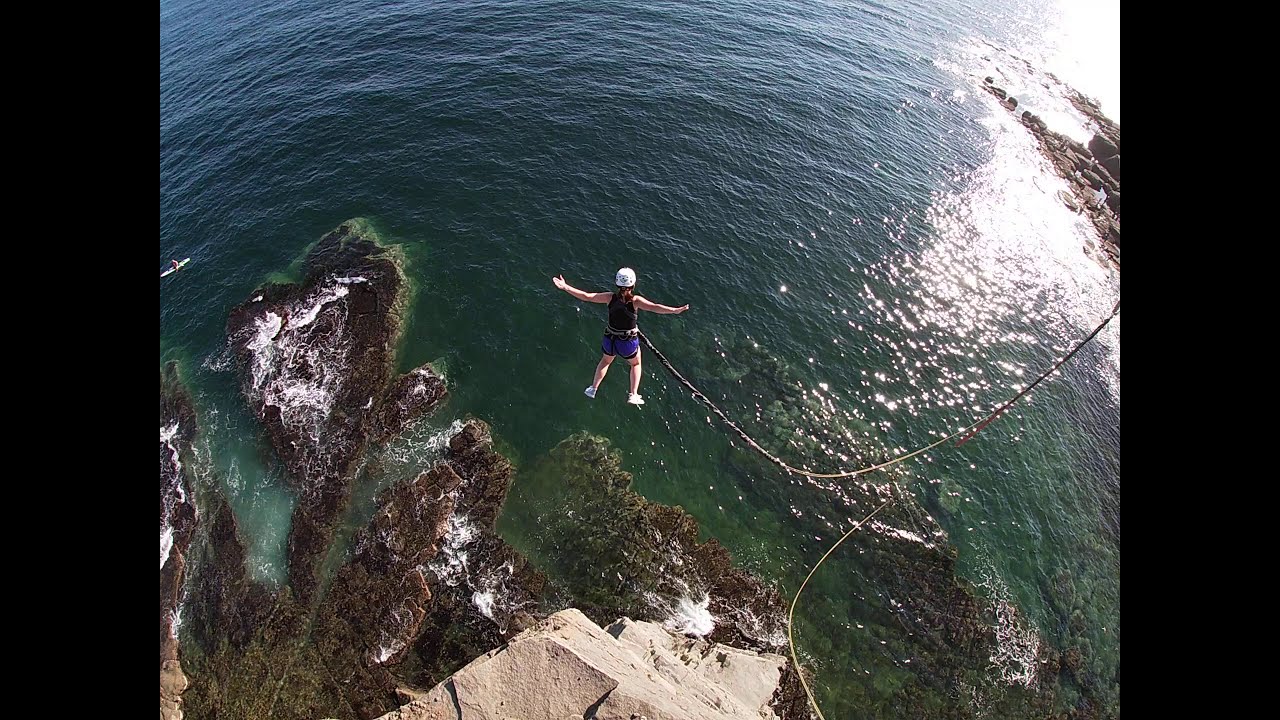In this breathtaking aerial image, a woman bungee jumps off a tan concrete platform on a rocky cliffside over a serene emerald green ocean. She is mid-fall, with her arms and legs outstretched in a slight spread, showcasing the thrill of the jump. The bungee cord, showing some slack, is attached to her right, ensuring she's securely connected. She is outfitted in a white helmet, black tank top, blue shorts, and white sneakers. The Sun in the top right corner casts a shimmering reflection across the calm, clear waters below, accentuating the vibrant greens and blues of the ocean. Rocks and a man-made jetty are visible along the right side, with waves gently crashing over them, adding texture to the scene. The reef beneath the water amplifies the stunning underwater landscape, completing this dynamic composition that captures both the excitement and beauty of the moment.